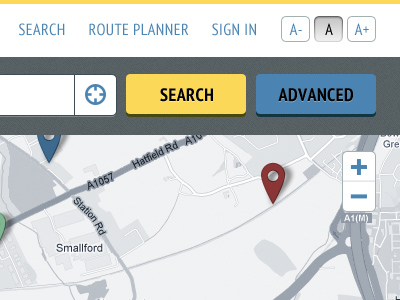The image depicts a detailed section of a web browser showcasing a web page interface. At the top, in the header area, there is blue text that reads "Search," accompanied by "Route Planner" and "Sign." These elements are aligned horizontally on the same line. Adjacent to these, there are three buttons for adjusting text size, labeled as "A-" on the left, "A" in the middle, and "A+" on the right. Below this header, there is a search bar meant for entering locations. This search bar features a yellow search button and a blue button labeled "Advanced," both with black text.

Beneath the search bar, a partially visible map displays specific elements, including labeled roads such as Station Road and an area called Small Ford. A crimson red waypoint marker is noticeable on the map. Additionally, plus and minus buttons are present, allowing users to zoom in and out of the map.